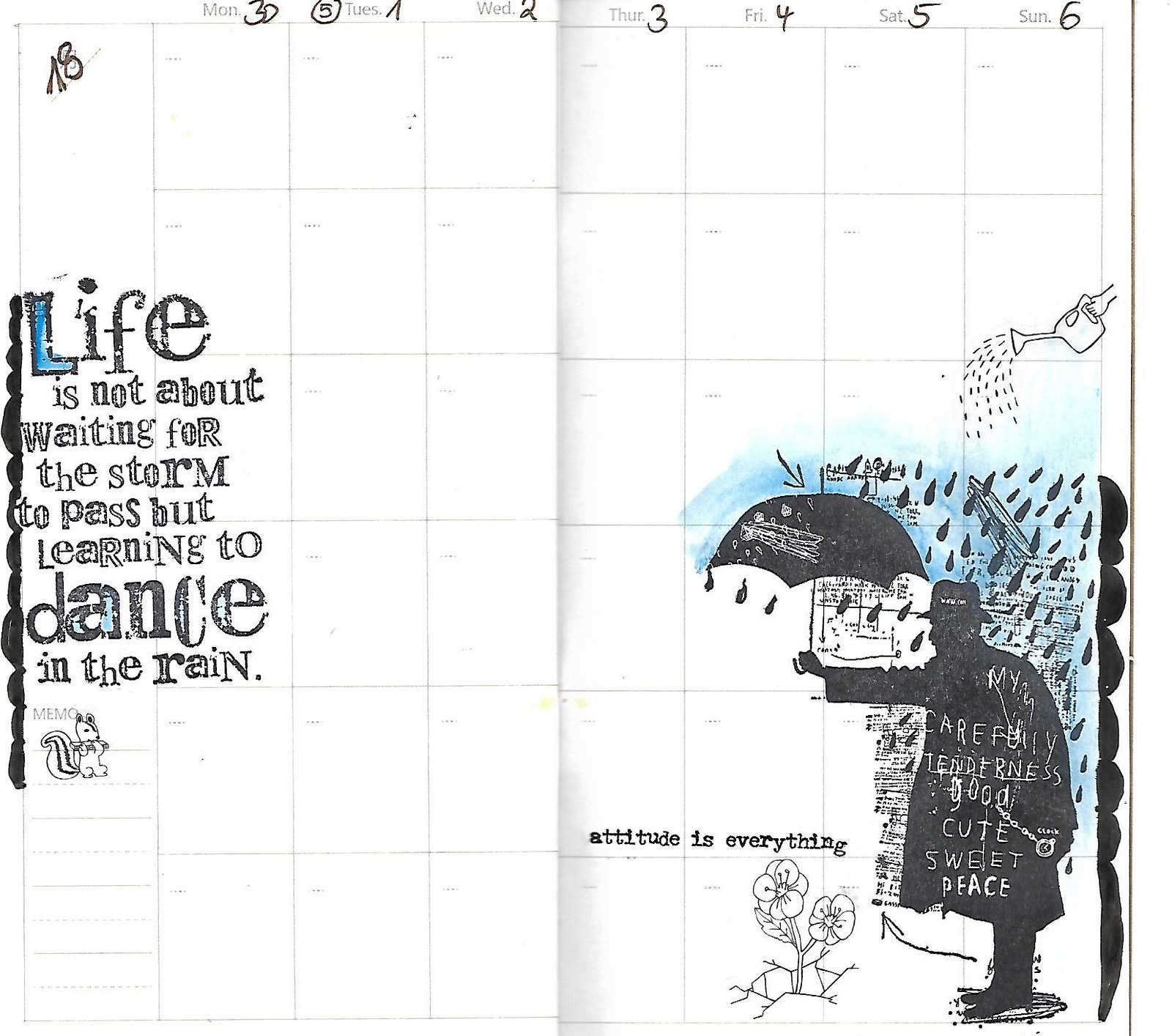The image is a creative, repurposed black and white calendar page designed as an artwork. The calendar grid spans from Monday to Sunday, with Monday labeled as the 30th, Tuesday as the 1st, Wednesday as the 2nd, Thursday as the 3rd, Friday as the 4th, Saturday as the 5th, and Sunday as the 6th. In the left margin, there is a stamped inspirational quote that reads, "Life is not about waiting for the storm to pass but learning to dance in the rain," accompanied by a tiny drawing of a squirrel beneath it. The L in "Life" is handwritten in blue. On the bottom right corner, there is a silhouette of a person wearing a trench coat and hat, holding an umbrella. This figure is being showered with black drops, symbolizing rain, and is protecting a flower. Carved into the silhouette are the words "carefully," "tenderness," "good," "cute," "sweet," and "peace." Above the character, the text "Attitude is Everything" is prominently displayed. The entire scene, including the person shielding the flower, emphasizes the importance of maintaining a positive attitude in challenging circumstances.